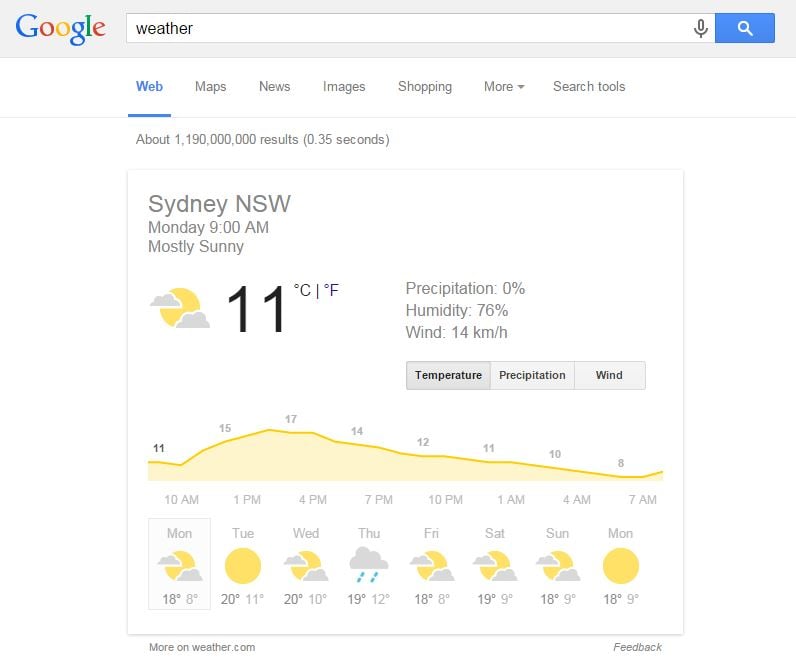The image displays a weather page from Google, focusing on the weather forecast for Sydney. At the top, the familiar Google logo is shown alongside the search bar on its right, which contains the current search query for weather. To the right of the search bar, there are the microphone icon and the search button. Just below this, you'll notice the various search categories including Web, Maps, News, Images, Shopping, along with options for More and Search Tools.

The search results indicate about 1 billion results found in approximately 0.35 seconds. The weather forecast details for Sydney show that on Monday at 9 a.m., it is mostly sunny with an average temperature of 11°C. The chance of precipitation is 0%, the humidity stands at 76%, and the winds are blowing at 14 kilometers per hour.

As the day progresses, the temperature is expected to gradually get colder. The forecast for Tuesday and Wednesday indicates similar temperatures with partly cloudy skies. There is a prediction of rain on Thursday. The weather from Friday to Sunday is expected to be cloudy, followed by a fully sunny Monday.